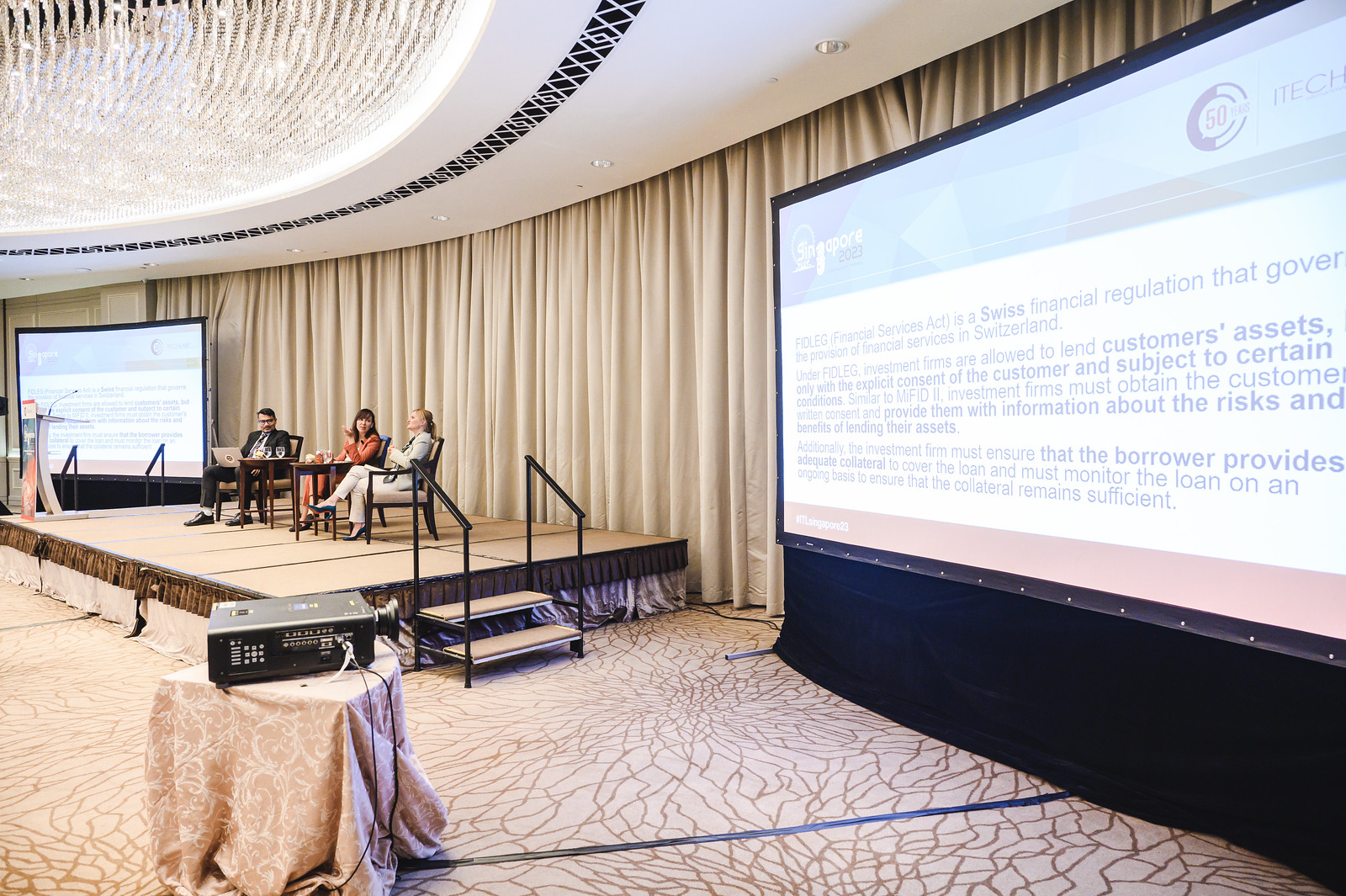The image captures a wide rectangular stage viewed from the side, centrally positioned on the left side. The light brown stage, not very high and with two steps leading up, features three individuals seated on wooden cushioned chairs. The leftmost individual is a man in a black suit with a silver laptop on his lap. In the middle is a woman in an orange suit, and to the right is a woman in a beige suit. Behind them stretches a beige curtain across the backdrop, with a white sequined portion in the top left corner of the ceiling above. The stage is flanked by two large screens displaying PowerPoints with blue logos at the top. The floor is multicolored in tan with black lines, and black masking tape is visible, marking the area to prevent tripping hazards, adding practical detail to the conference room setting.